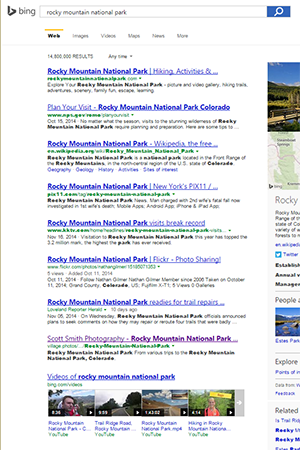This is a detailed screenshot of a Bing search results page. In the top left corner, the Bing logo is prominently displayed next to the search engine's name. Adjacent to this on the right is a search bar, which features a blue search button at its end. Beneath the search bar, a menu bar offers various search categories: Web, Images, Videos, Maps, News, and More. A yellow line above the "Web" category indicates it is currently selected.

The search results page is populated with numerous links, specifically displaying eight links in this view. The first link directs to "Rocky Mountain National Park Hiking Activities". Following this, the second link offers information on "Plan Your Visit to Rocky Mountain National Park, Colorado". The third link leads to the Wikipedia page for "Rocky Mountain National Park". Additional links are listed, with the final one marked as "Scott Smith Photography, Rocky Mountain National Park". This last link has been previously clicked, thus appearing in purple instead of the default blue.

Below these links, there is a section dedicated to videos related to Rocky Mountain National Park, displayed in a horizontal slider featuring four video thumbnails. To the right of the video section, a truncated embedded map accompanies some images, although this portion is partially cut off in the screenshot. Additionally, there is a section for reviews, along with topics related to the search and suggestions for what other people have searched for.